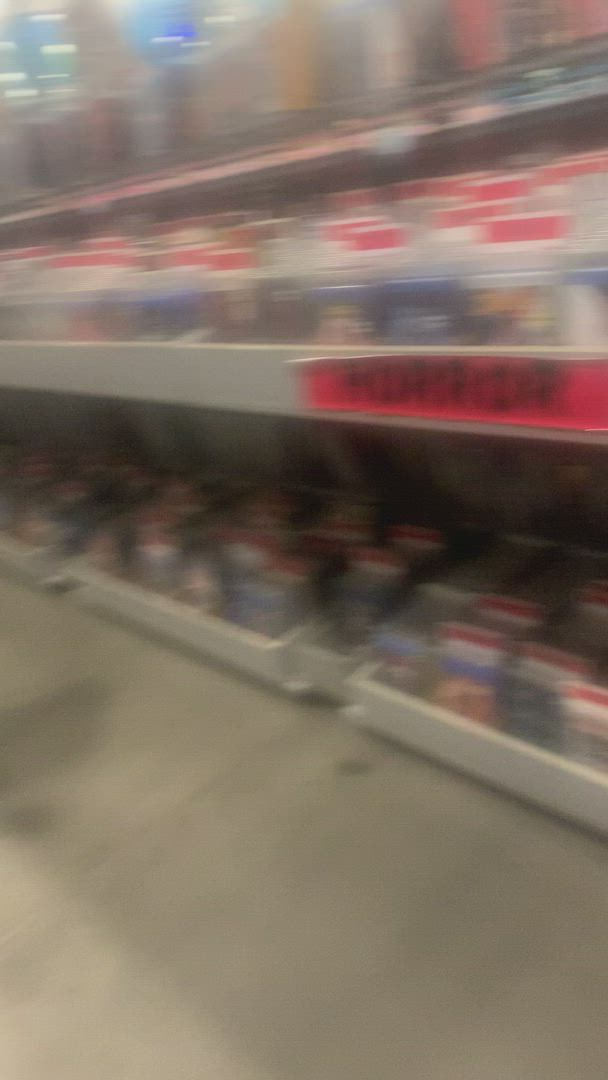The image appears to be an extremely blurry, low-quality photograph taken inside a store, possibly a bookstore or a movie rental shop. The horizontal motion blur and a foggy, smudged lens give the scene a brownish tint. This long portrait-style image captures two sections of shelves that are likely holding books or magazines. Each item on the shelves features a red rectangular stripe at the top, and the labels appear to be indicating a genre, with one visible label reading "horror." The shelves are positioned above a smooth, gray concrete floor, which is also blurred. At the bottom of the shelves, items—potentially magazines—are lined up, displaying mostly blue covers with white and red stripes. The image also shows a neon magenta sticker with illegible lettering on the front edge of the top shelf towards the right side. Overall, the scene evokes a nostalgic vibe reminiscent of old video rental stores like Blockbuster.